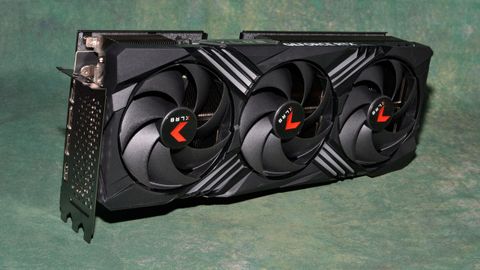The image features a detailed, horizontally oriented assembly of three fans, often used in PC builds. Each fan is centrally positioned within a larger structure, with one fan in the middle, one to the right, and one to the left. The fans are enclosed within this framework, showcasing a combination of black, gray, and red colors in their design. The background of the image is a distinctive seafoam green, which appears uniformly across the entire backdrop, possibly suggesting it was digitally added. The image has a modern aesthetic, comparable to that of a contemporary boom box, with a sleek, plasticky appearance. The focus of the photograph is primarily on the central trio of fan blades, which are depicted at a slight angle from front left to back right, enhancing the depth of the composition.